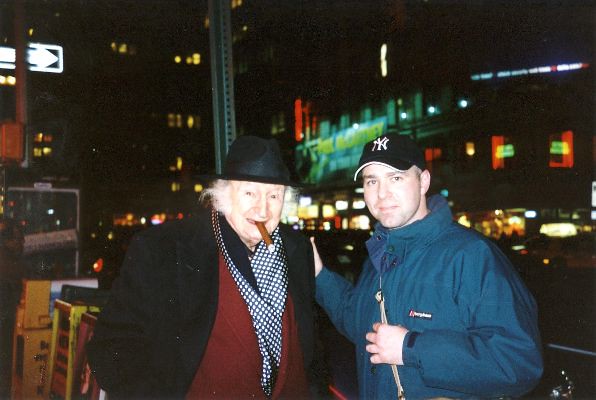The photograph captures two men standing against an urban night backdrop with illuminated buildings and numerous cars lining the streets. The first man, presumably older, stands on the left, distinguished by his distinct white bushy hair and jovial, toothless grin. He is adorned in a dark hat, alongside layered clothing consisting of a black jacket over a red one, complemented by a white polka-dotted black shawl draped around his neck. A notable detail is the large brown cigar he is smoking. To his right stands a younger man, sporting a blue winter coat and a black baseball cap with a distinctive white New York logo pattern. A backpack strap runs diagonally from his right shoulder to his left thigh, adding to his casual look. Despite the vivid street and building lights, the exact location remains indistinct.